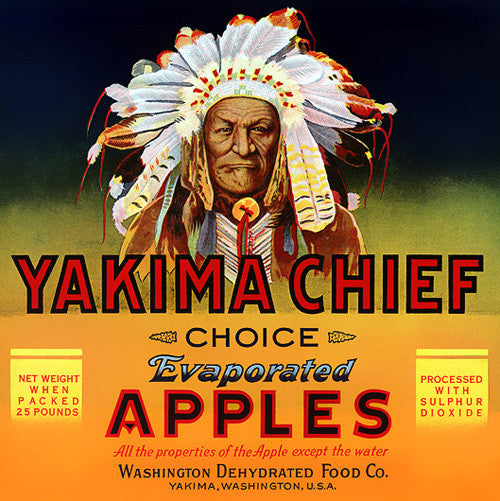The poster is an advertisement for Yakima Chief brand evaporated apples, produced by the Washington Dehydrated Food Company, Yakima, Washington, USA. At the top of the poster, there is a detailed illustration of an older Native American Indian chief wearing a traditional feather headdress and a choker. His face is etched with wrinkles that accentuate his stern expression. Below this striking image, in bold red lettering with a black outline, the words "Yakima Chief" are prominently displayed. Beneath this in an orange box, the text reads "Choice," followed by "Evaporated" in blue, and then "Apples" in black with a red outline. The caption "All the properties of apples except for the water" explains the product’s attributes. Further down, the text provides logistical details, such as "Washington Dehydrated Food Co, Yakima, Washington, USA" and "Net weight, when packaged, 25 pounds" on the left. On the right side, it is noted that the product is "Processed with sulfur dioxide." The background of the poster transitions from black at the top to green and then to orange at the bottom, framing the vibrant and detailed typography and artwork.